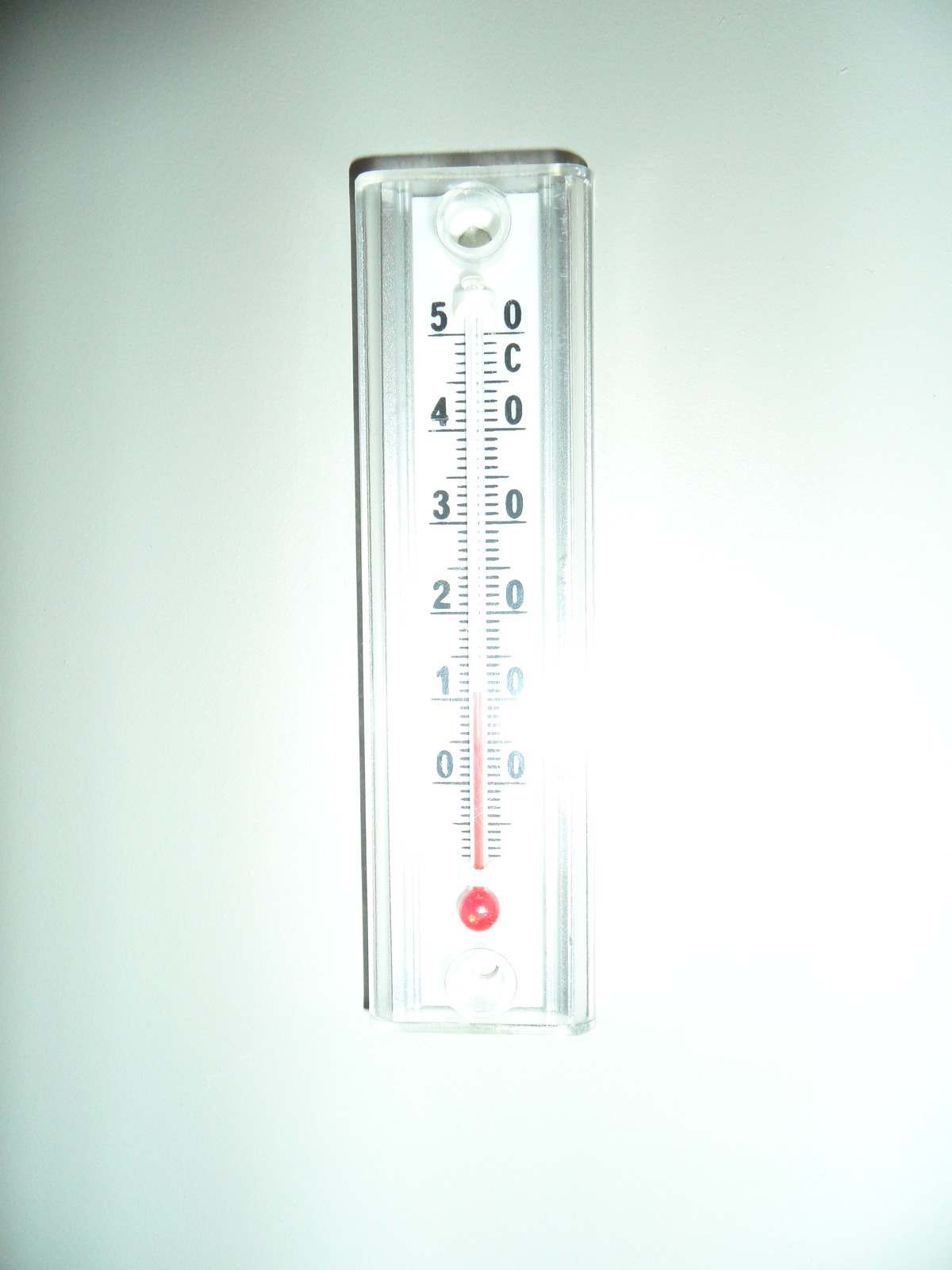In this vibrant color photograph, a classic thermometer lies against a light blue background, bathed in bright light that slightly overexposes the image. The thermometer, a long rectangular object made of clear, see-through plastic, features precise gradations in both Celsius and Fahrenheit. The Celsius scale, located on the right side, ranges from 0 to 5 degrees, each marked in black against a pristine white backdrop. Below the zero mark, a distinctive little red circle catches the eye. Climbing from this point is the red mercury, prominently visible through the center of the scale, indicating a temperature around 0.5 degrees Celsius. Meanwhile, the Fahrenheit scale on the left side curiously displays only zeros. Adding to the intrigue, the top of the thermometer features a small circle, whose function remains unclear, adding a touch of mystery to this otherwise scientific instrument. The overall composition, with its precise details and a hint of overexposure, gives the thermometer a surreal, almost abstract quality.